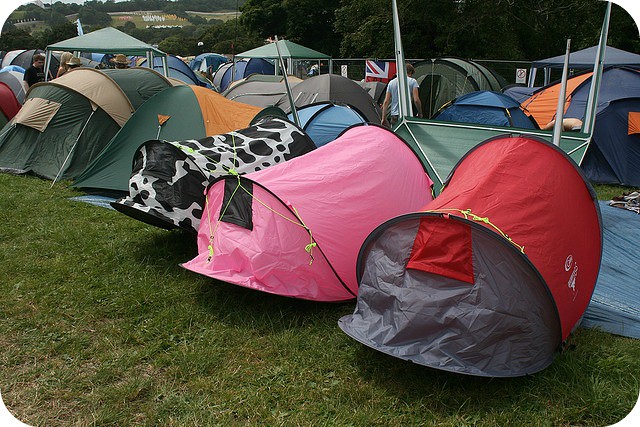The image depicts a vibrant camping site adorned with an array of colorful tents scattered across lush green grass. The colorful tents range from red, pink, and green, to more unique designs such as a tent with black spots on a white background, resembling a cow's print. Among the clearly visible tents, the rightmost one is red, while another nearby tents are pink and multicolored. In the midst of the campsite, a flag from Great Britain stands out prominently. Throughout the scene, campers are seen walking around and mingling among the tents, enhancing the lively atmosphere. The bright daylight illuminates the whole area vividly. In the background, to the upper left, towering mountains and an expanse of verdant trees complete the picturesque outdoor setting.